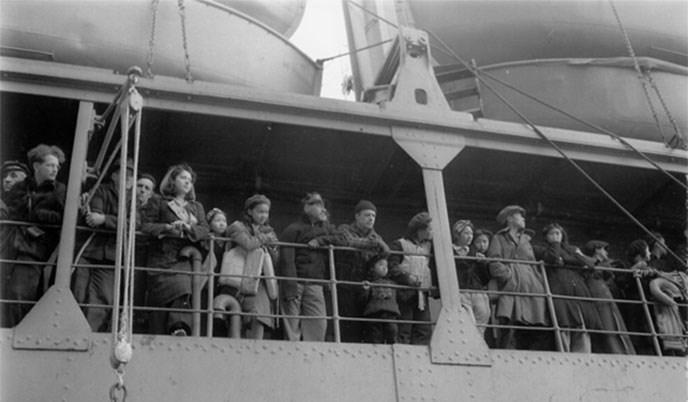In this vintage black and white photograph, a large group of people, ranging from children to older adults, is seen standing and leaning against a guard rail on the edge of what appears to be a steel-based boat or dock. The image is shot from a slightly lower angle, looking up at the individuals. They are all dressed warmly in winter clothing, including long pants, long-sleeve jackets, and hats, suggesting a cold environment. Visible above the group are two large, concave metal structures, along with beams extending from the roof to the base of the structure, adding to its industrial appearance. The people, who seem to be of various races, are facing outward, possibly looking at the water or the shore, although the exact scenery remains unclear. The overall setting and attire suggest that the photograph was taken around the 1940s or 1950s.